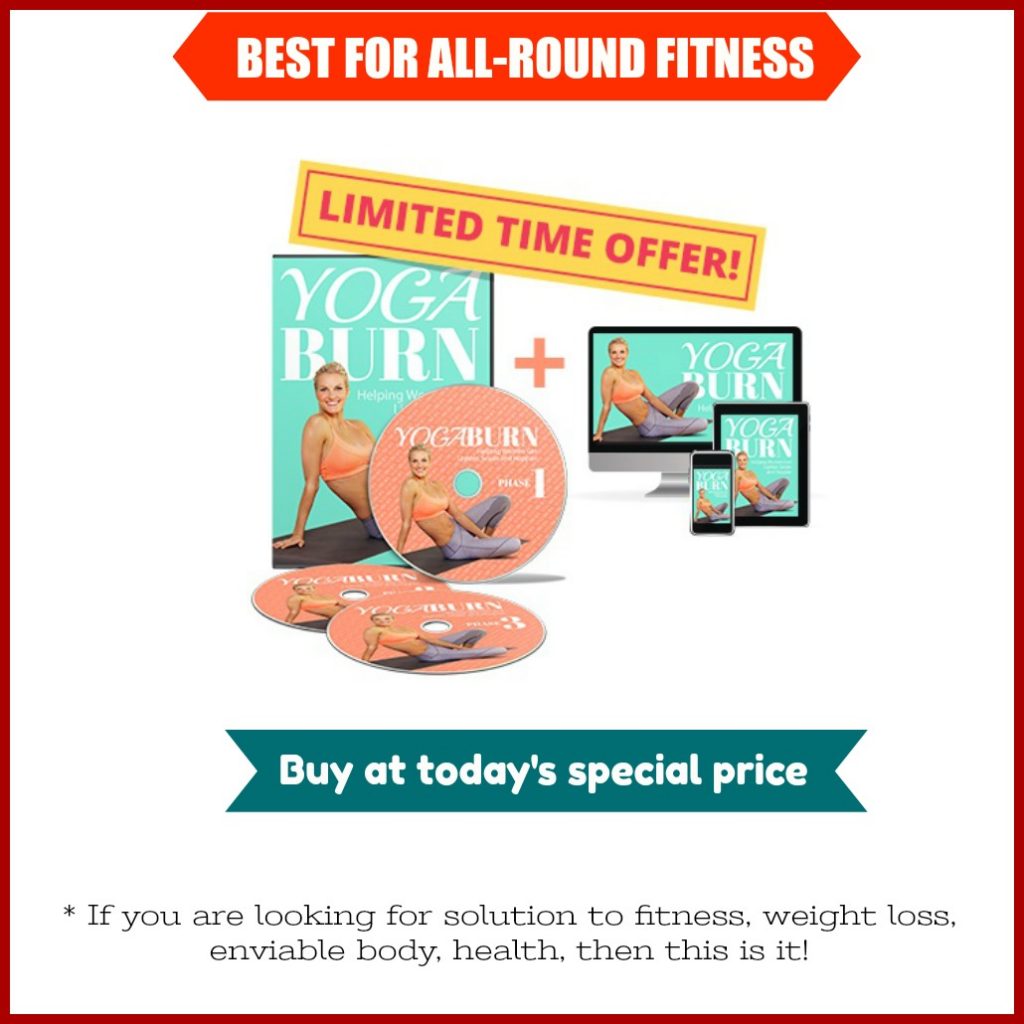Here's a cleaned-up and detailed caption for the image described:

---

The advertisement promotes the "Yoga Burn" fitness plan, showcasing it as ideal for all-round fitness. The top of the ad features a banner with pointed ends resembling a dual-direction sign, highlighting in bold white font on a red background, "Best for All-Round Fitness."

Central to the ad is an array of products included in the Yoga Burn bundle. At the center, there's a DVD package set against a vibrant turquoise background, prominently displaying the "Yoga Burn" branding. Featured on the cover is an image of a woman wearing a coral or salmon-colored sports bra and gray yoga pants. She is seated somewhat awkwardly on a black yoga mat. This image is consistently used across all Yoga Burn products, including the DVD cover, the individual discs, and the app interfaces.

The discs themselves are pink and labeled with the same Yoga Burn image along with text indicating different phases of the program, such as "Yoga Burn Phase 1," "Phase 2," and "Phase 3." These discs are positioned in front of the DVD cover, clearly shown within the bundle. Adjacent to this, a plus sign and the word "Yoga" are prominently displayed, emphasizing the program's comprehensive approach.

Additionally, the ad features digital devices including a Mac computer, an iPad, and an iPhone, all displaying the Yoga Burn interface in the signature teal background with the same image of the woman on the yoga mat.

Above these elements is a yellow rectangle bordered with inset red, containing the text "Limited Time Offer" in bold red font. Below this, a ribbon banner reads "Buy it today's special price" in white font. Further down, another message in black font states, "If you are looking for a solution to fitness, weight loss, enviable body health, then this is it."

The entire ad is framed with a bold red border, encapsulating the promotional message and products within it.

---